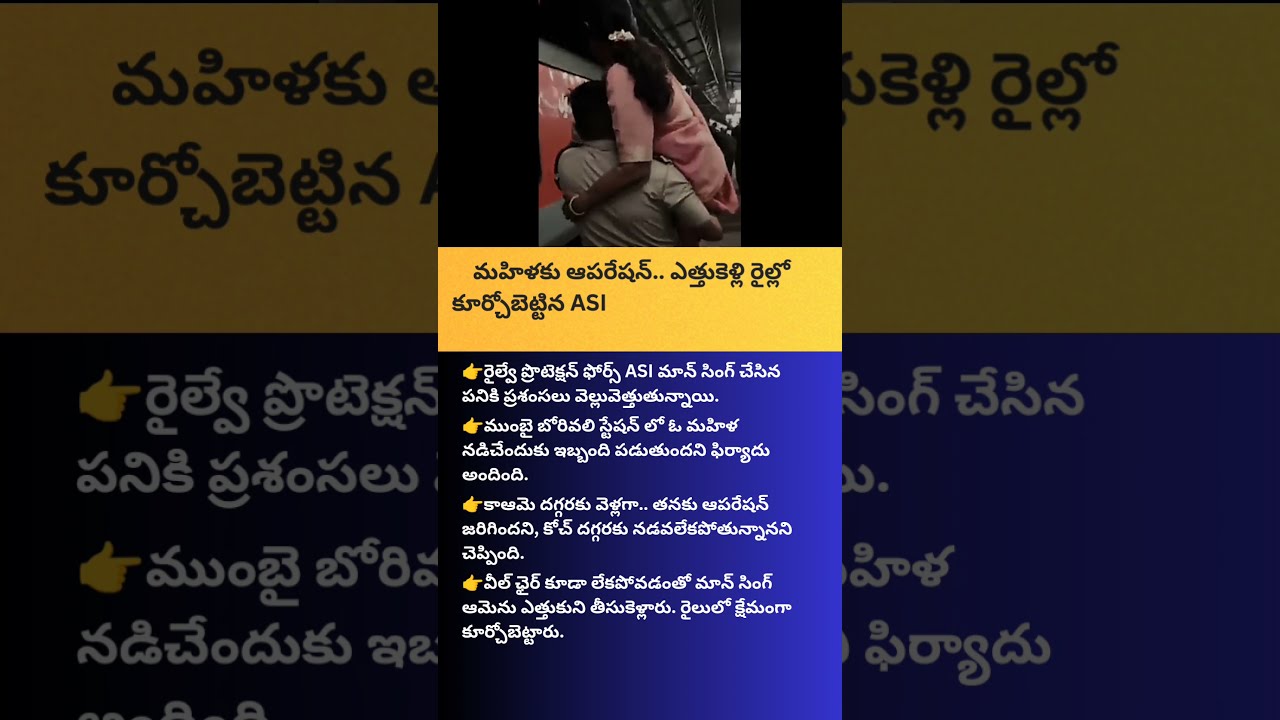In this horizontal, rectangular image, set against a backdrop of a faintly darkened graphic that is slightly enlarged, we see a central picture featuring a man and a woman in what appears to be a Middle Eastern setting, possibly a train station or an outdoor scene at night. The couple, captured from the back and mid-torso up, shows the man carrying the woman. He has short black hair and wears a gray or off-white shirt, while the woman, with her long black hair pulled back into a fluffy ponytail, is dressed in pink and has her arm wrapped around him.

The top portion of the image is highlighted by a dull yellow horizontal rectangle containing text in a Middle Eastern language written in a dark blue or black font. Below this, dominating the bottom half of the image, is a dark blue rectangular area with white Middle Eastern script. Four yellow hand emojis point towards different lines of text, emphasizing each section. The background details are partially obscured but show a zoomed-in, shaded view of the same image and script, tying the whole composition together in a layered, visually rich style.